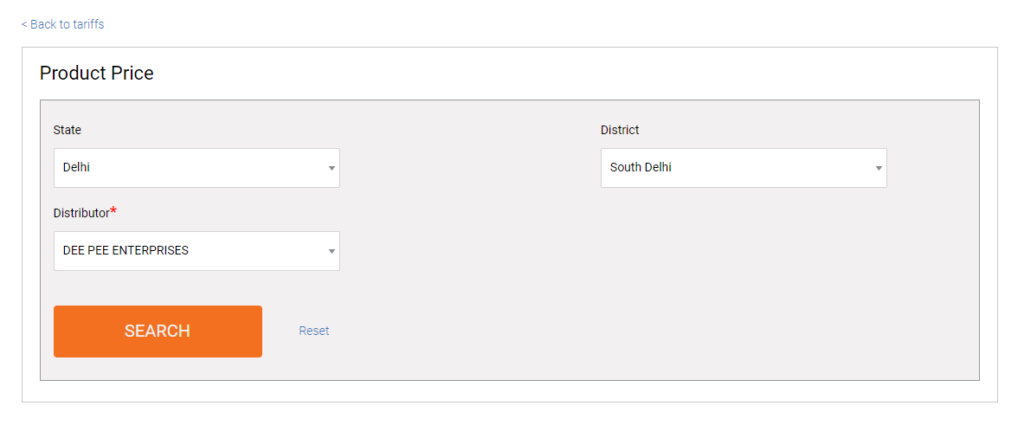The image appears to be a user interface from a website, likely related to tariff or product pricing adjustments. The interface includes a main section for user inputs and selections.

At the very top left corner of the page, there is a navigational link labeled "Back to Tariffs" accompanied by a left-arrow symbol, both rendered in blue text. This link is located just above the primary input section.

The central part of the interface is dominated by a large white box encompassing a slightly smaller gray box within it. In the top left corner of the white box, the title "Product Price" is prominently displayed, indicating the purpose of this section.

Within the gray box, situated at the top left, there's a label reading "State," adjacent to a drop-down menu currently set to the option "Deli." Below this, there's another label for "Distributor," marked with an orange asterisk to denote a required field. This drop-down menu is currently set to "DP Enterprises."

At the bottom left corner of the gray box, there's an orange "Search" button for submitting the inputted information. To the right of this button, in small blue text, lies a "Reset" option for clearing the selections.

In the top right corner of the central white box, the label "District" is specified, with "South Deli" selected from its drop-down menu.

The labels for "Category," "State," "Distributor," and "District" are positioned outside the main white box, written in smaller text, while the corresponding drop-down selection options lie within the white box, providing areas for user interaction and selection.

This interface segment is well-structured to guide users through selecting product pricing details, distributor information, and other relevant data points essential for tariff management.